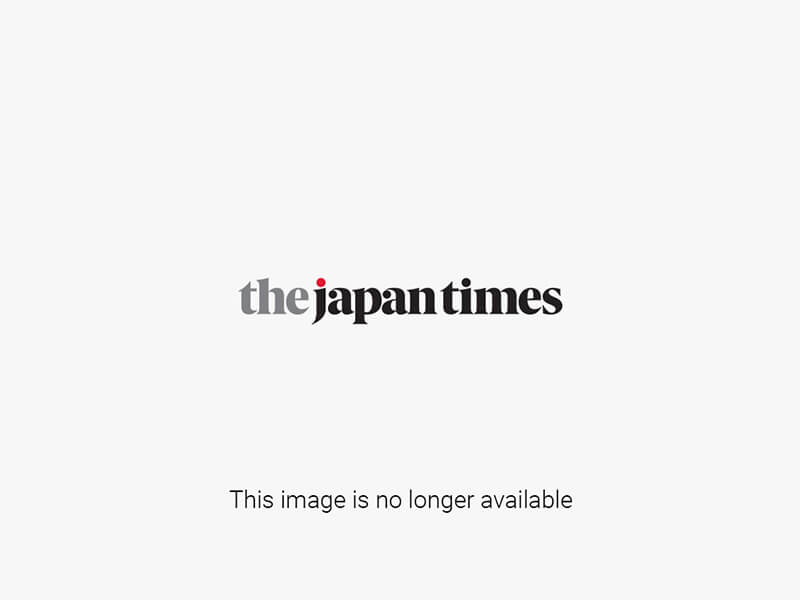The image features a set of three Japanese yen banknotes, arranged vertically against a plain black background. Each banknote bears the word "specimen" in red and black stamps.

At the top is the ¥10,000 note, which showcases a Japanese man in a black suit on the right side, who is looking directly forward. The left side of this note transitions from an orange color to blue, then greenish-yellow, and ends in red. There's a large white circle with a red and black speciment stamp diagonally across it, saying "specimen" in large red letters and twice in smaller black letters. Additionally, the note displays the denomination of 10,000 on the top left and lower right corners, accompanied by the text "AA 900 198 AA" and "Bank of Japan," as well as a red circle with Japanese writing.

In the middle, the ¥5,000 note features a woman in a kimono with her hair up in a bun, facing slightly to the left. The background of this bill shifts from purple on the left to blue in the center and back to purple on the right. The woman is positioned on the right side, with the denomination of 5,000 on the top left and lower right corners, alongside the serial number "AA 900 198 AA," and the text "Bank of Japan." This note also includes the red circle with Japanese writing beneath the main text.

At the bottom is the ¥1,000 note, presenting a man with a mustache and small glasses, dressed in a suit with a bowtie, on the right side. The background starts and ends with light blue and contains a central yellow-orange hue. Similar to the other notes, it has the denomination of 1,000 on the top left and lower right corners, the serial number "AA 900 198 AA," and the text "Bank of Japan" with the accompanying red circle with Japanese writing. A small image of the man's face is also found in the lower left corner. There is a white oval with a red and black speciment stamp reading "specimen" once in red larger letters and twice in smaller gray letters.

Each banknote features an intricate and colorful design, marked as specimens by the text "specimen" stamped three times on each note.